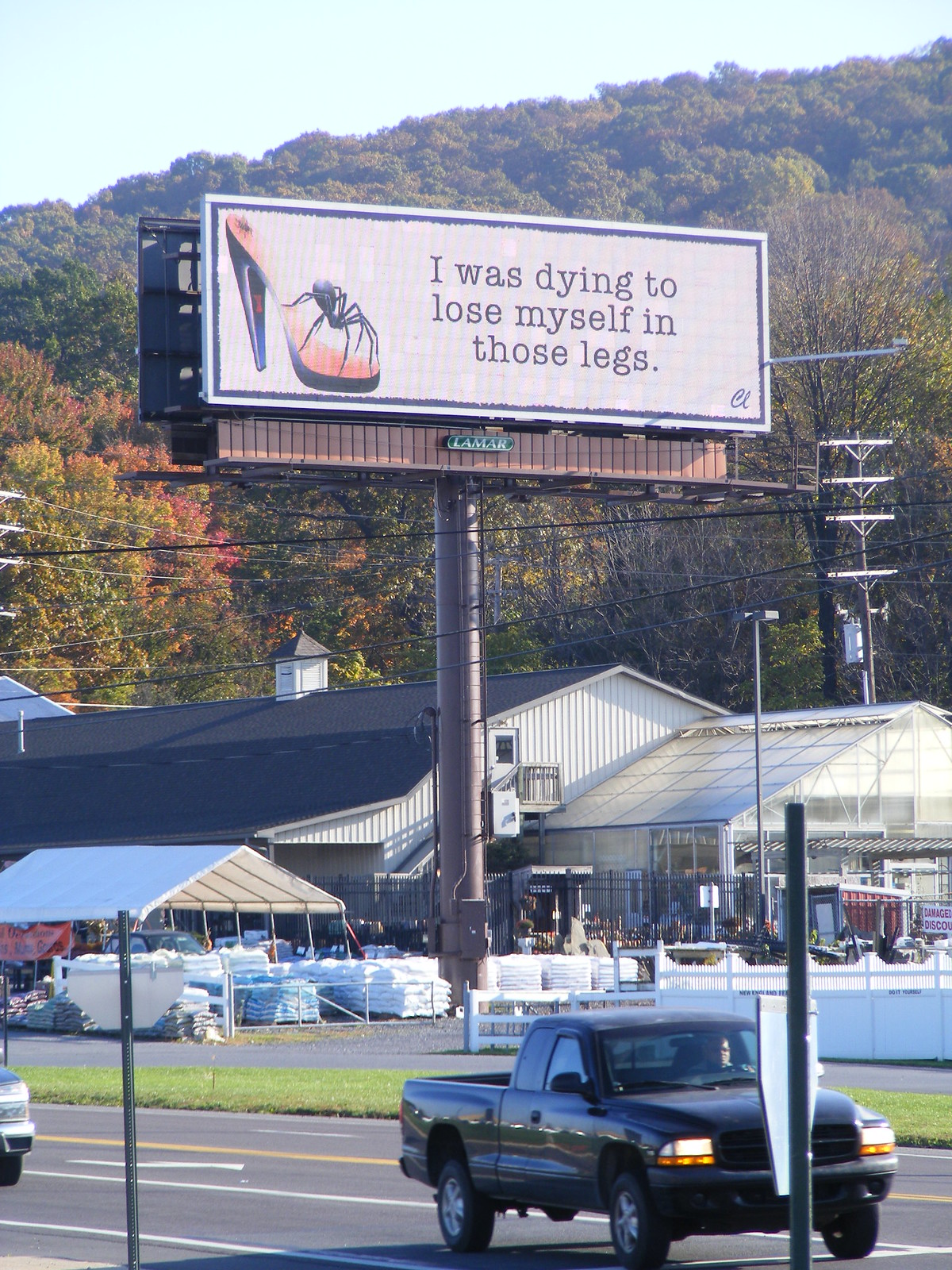The image depicts a bustling scene at a large garden center situated in a rural area, against the backdrop of an enormous hill and verdant trees just starting to turn to autumn hues of orange and yellow. Dominating the scene is a prominent billboard, mounted on a thick brown metal pole near the entrance, with the mysterious phrase, "I was dying to lose myself in those legs,” accompanied by an image of a high-heeled shoe with a spider perched on the front. Below the billboard, a black Dodge pickup truck moves along the road, with the bumper of another vehicle visible nearby. The garden center itself is expansive, featuring a tent with various bags, a greenhouse, and a central store stocked with items for lawn and farm care. Electrical wires run across the sky, framing the scene and adding to the rural yet industrious ambiance.